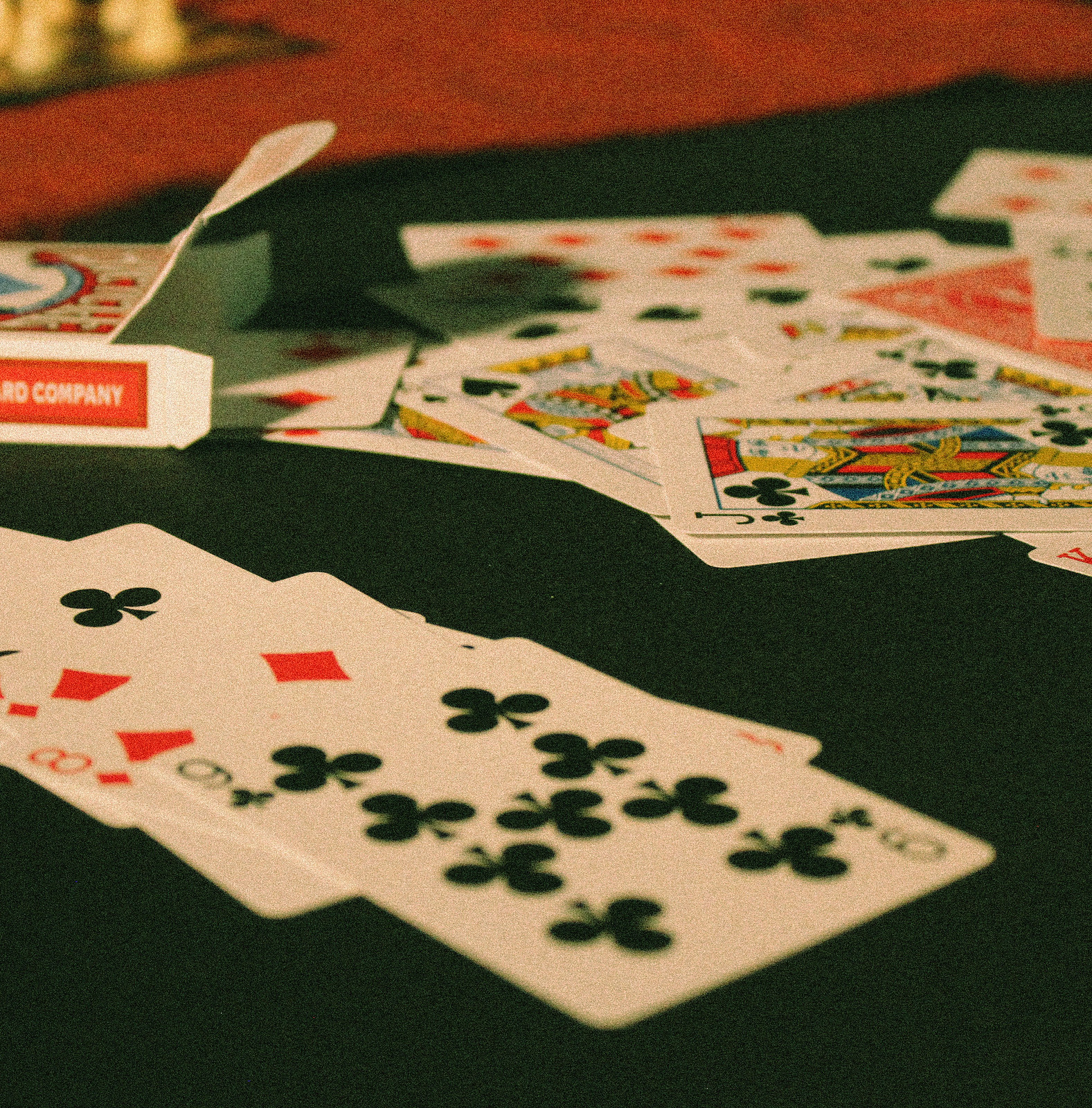This photograph exudes an almost professional quality, possibly enhanced with a textured, pixelated filter that adds a unique visual effect. The image is dimly lit, focusing on a green felt card table. In the upper left-hand corner of the table lies an open, white cardboard box adorned with red graphics; it is partially out of the frame, spilling a chaotic array of playing cards across the surface. Dominating this disordered pile, the King of Spades and the Jack of Clubs are prominently visible. Additionally, a neat row of cards extends from the lower left to the lower right corner of the table. In this row, one card is partly cut off, next to an 8 of Diamonds, with a 9 of Clubs lying above it. All these elements rest upon the green felt surface, contributing to the scene's overall disheveled yet captivating ambiance.